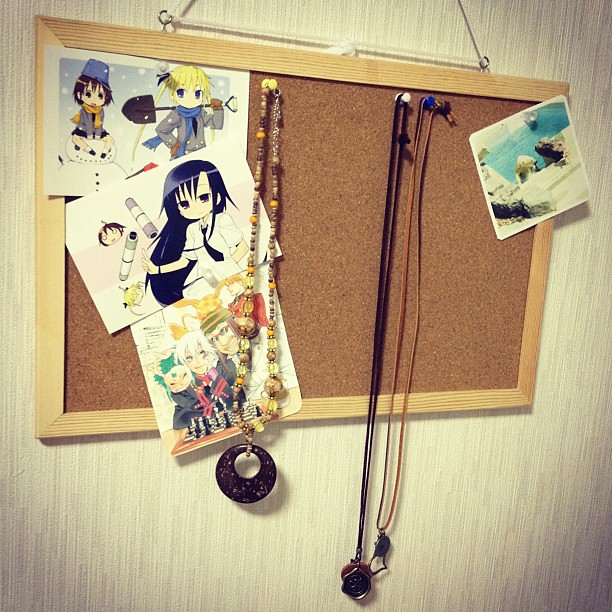This is an image of a cork bulletin board with a wooden frame, hanging on a light gray, textured wall with a string forming a triangle at the top for support. On the left side of the board, there are three anime-themed pictures arranged vertically in a slightly tilted manner. The topmost anime character has blonde hair, wears a gray jacket with a blue scarf, and holds a shovel. Below this, another character has long black hair and a black tie. The last image in this sequence shows a series of animated characters in a group hug from a frontal viewpoint.

Adjacent to these pictures hangs a necklace from a yellow pushpin. This necklace features a large black circular pendant with a hole at the top. Another necklace dangles from a white pushpin, characterized by a black string holding a dark circular pendant. A third necklace, attached to the board by a blue pushpin, has rawhide elements and a dark metal emblem. In the upper right corner of the bulletin board, slightly askew, is a photograph of an outdoor beach scene. It shows an expanse of blue water surrounded by white cliffs, fastened with a clear pushpin.